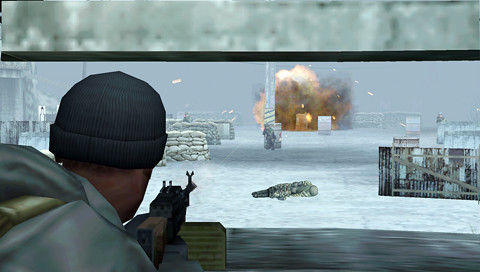In this still from a mid-2000s era video game, reminiscent of "Counter-Strike," a black man is depicted in a tense moment within a bunker environment. The game appears to be a first-person or third-person shooter. The character has just fired at a canister, causing an explosion that illuminates the scene. The overall visual quality is not high-definition, characteristic of games from that period, and the frame is dominated by white and greenish hues. The scene captures the gritty and suspenseful atmosphere typical of early action shooters.